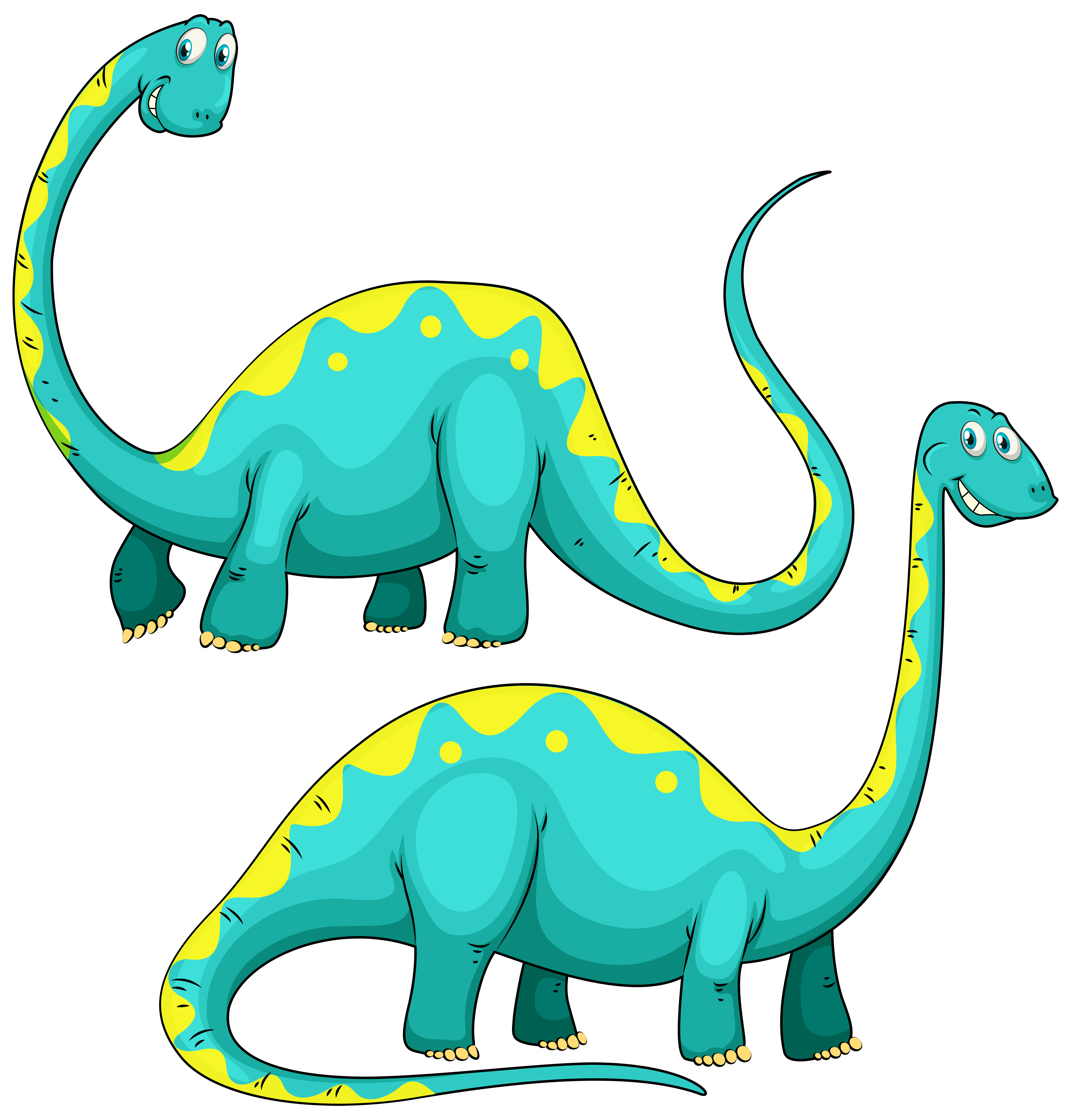The image features two cartoonish dinosaurs rendered in shades of teal and featuring bright yellow accents. Both dinosaurs have elongated necks and tails, with a slightly humped back. They are decorated with a lime green scalloped stripe running from near their heads all the way down their backs to their tails. Additionally, each dinosaur has three yellow polka dots aligned along their spines.

The dinosaur positioned at the top of the image is facing the left with its head turned back to the right, displaying a cartoonish smile and its visible teeth. The dinosaur at the bottom is oriented to the right, also looking back slightly, and is similarly smiling. Both dinosaurs have four limbs, each with five yellow toes. Their eyes are drawn with black pupils that enhance their expressive appearance. The tail of each dinosaur ends in a sharp point and is rendered in a darker teal shade. The overall color palette includes dark teal, medium dark teal, and light teal, with the yellow details adding vibrant contrast.